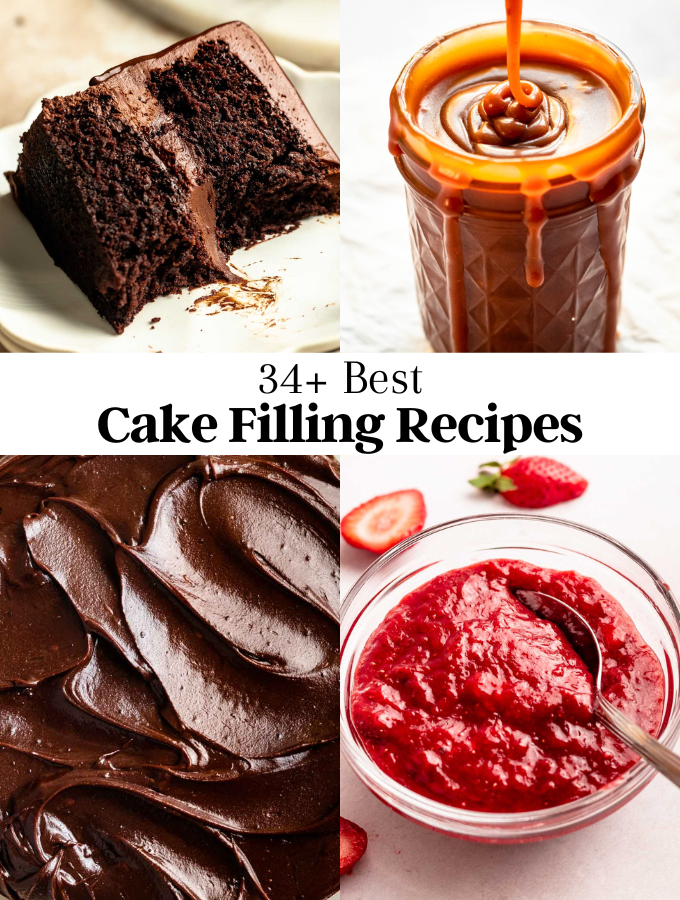This image is a collage composed of four distinct food photos arranged around a central white bar that reads "34 Best Cake Filling Recipes" in bold lettering. 

The top left section features a partially eaten slice of chocolate cake, possibly accompanied by ice cream. Directly to the right of it, in the top right corner, is a jar overflowing with a thick, caramel-like substance. 

In the bottom left corner, there is a close-up of chocolate icing, spread smooth and glossy over an unidentified surface. Finally, the bottom right quadrant shows a jar brimming with vibrant red strawberry sauce with sliced strawberries scattered nearby.

Each section collectively showcases different cake fillings and toppings, contributing to the comprehensive theme of the image.